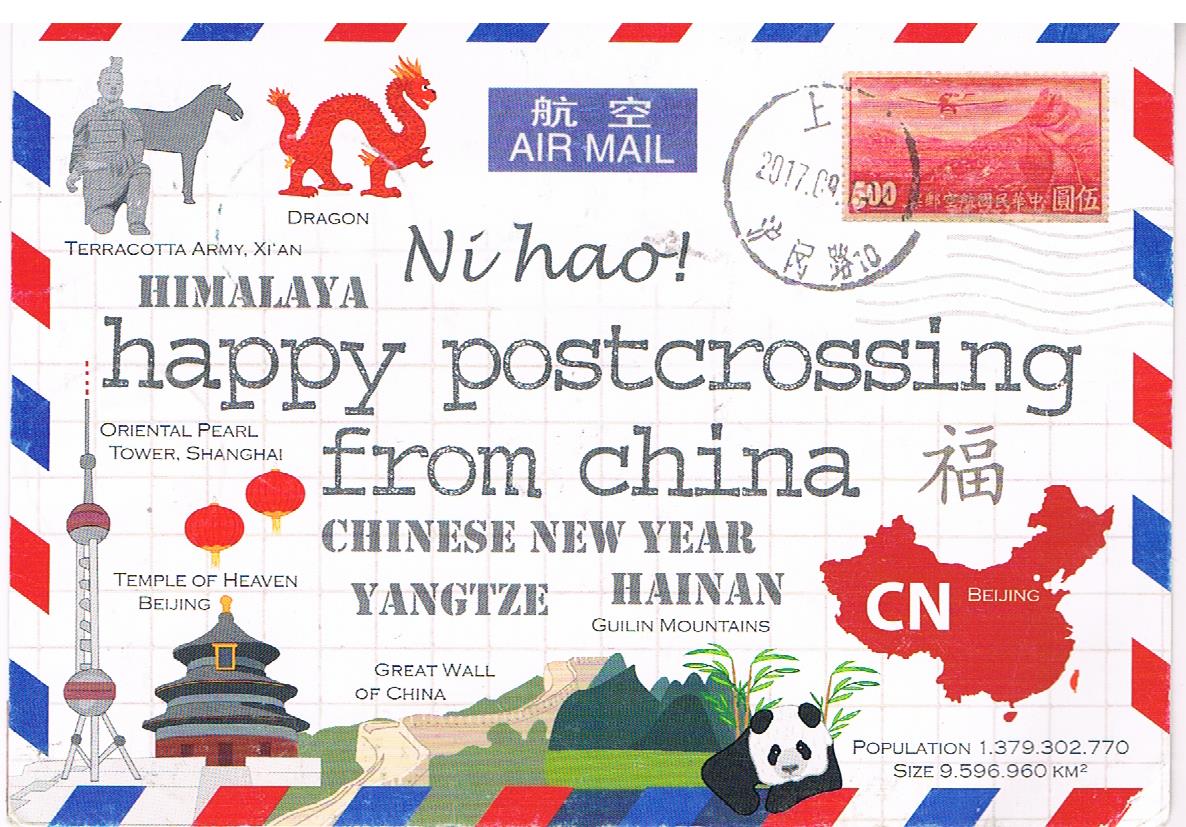The image showcases the front of an envelope adorned with a multitude of distinct details that lend it a rich and festive character. In the top right-hand corner, a red rectangular stamp is prominently displayed, indicative of its postal journey. Just below it, the blue label with the words "Air Mail" confirms its international dispatch. The top left-hand corner features an intriguing illustration of a kneeling man, a horse behind him, and a vivid red dragon adjacent to the horse.

Amidst an array of different fonts and sizes, the top of the envelope boasts an eclectic mix of text. It warmly greets with "Ni Hao" and goes on to name numerous iconic Chinese landmarks and elements, such as "Himalaya," "Yangtze," "Hainan," "Guilin Mountains," "Great Wall of China," "Temple of Heaven, Beijing," "Oriental Pearl Tower, Shanghai," and "Terracotta Army." These words encapsulate the essence of Chinese geography and cultural heritage.

In the bottom right-hand corner of the envelope, there is a red depiction of China with the word "Beijing" prominently featured. Underneath, there are references to population and size, further adding to the envelope's informative nature.

Finally, the envelope's celebratory note is encapsulated in the repeatedly mentioned phrase "Happy Post Crossing from China," which resonates across the image, creating a sense of joyful connectivity.